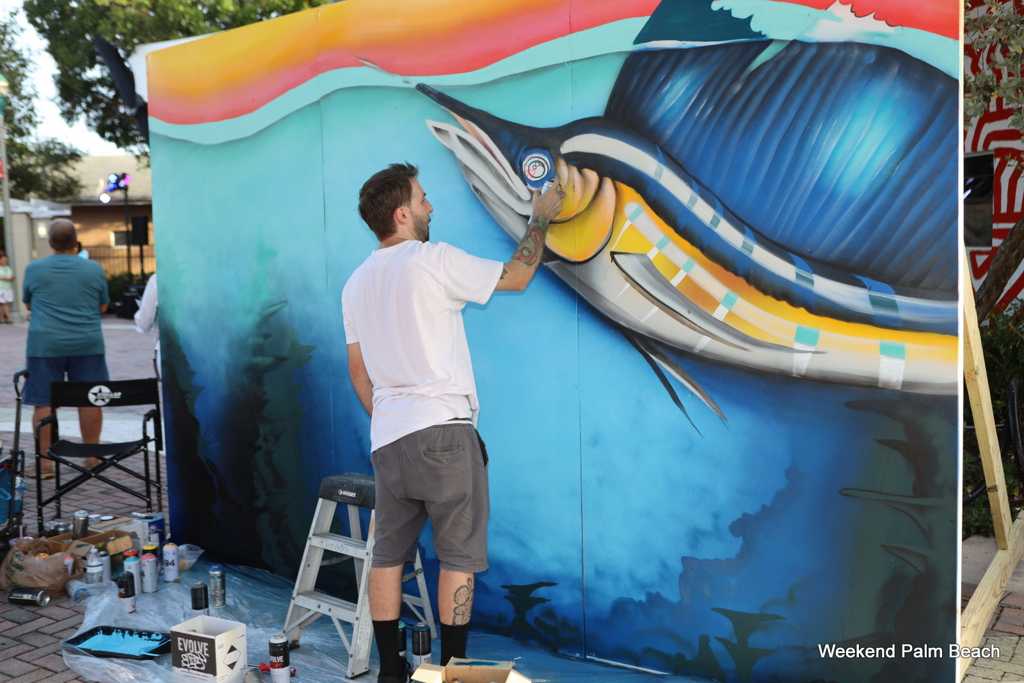In a vibrant outdoor setting, a dedicated white man with short brown hair and a beard stands before a large, upright canvas, painting an intricate mural of a swordfish. Clad in a white t-shirt and slightly sanded black knee-length denim shorts, he meticulously works on the detailed artwork which features a blue-scaled fish with shades of yellow and blue stripes, silver fins, and a prickled nose. The swordfish is set against a background that transitions from dark blue at the bottom to light blue at the top, accented with waves of pink, yellow, and orange. The scene is framed with a hint of sky and trees in the upper left corner.

In the foreground, a light blue paint vesicle sits among various beverage cans and plastic wrap spread over the ground to protect the pavers. A nearby two-step folding metal ladder with a black top provides the artist with necessary reach. Adjacent to the mural, an older person wearing a green shirt and blue shorts stands with their back to the camera, partially visible. The photograph, labeled "Weekend Palm Beach" at the bottom, captures the essence of an open-air event, showcasing the artist's process amidst a casual yet detail-oriented atmosphere.